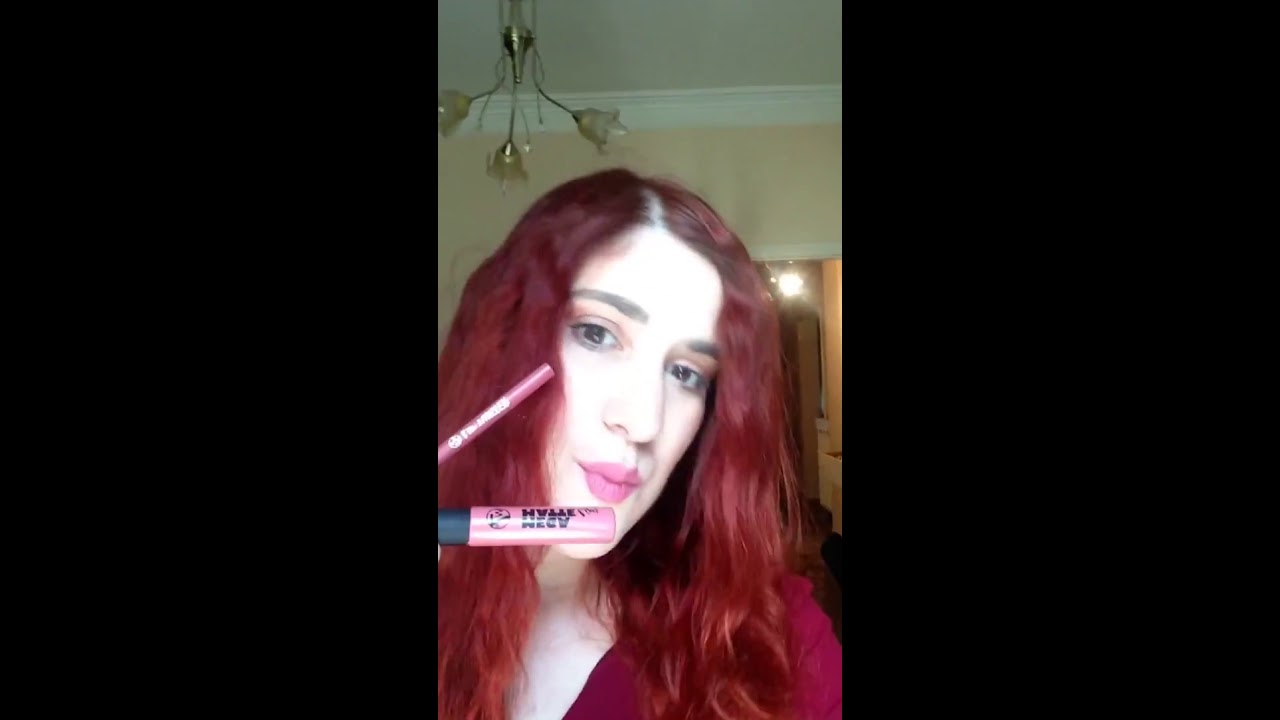The photograph features a girl with very pale, white skin and wavy, bright red hair, sitting close to the camera in her room, which appears to be part of a home or apartment. She has a distinctive pouty lip expression as she showcases her makeup products, holding up a pink lipstick tube and a raspberry-colored lip pencil that complement her pink lips. Her manicured dark brown eyebrows and brown eyes accentuate her attractive, elongated face. Dressed in a maroon, raspberry, or pink shirt, she creates a striking contrast that highlights her cosmetics. Behind her, the room’s light cream walls, white ceiling, and a chandelier with golden lamp covers and light yellow light bulbs are visible, contributing to the warm lighting of the scene.